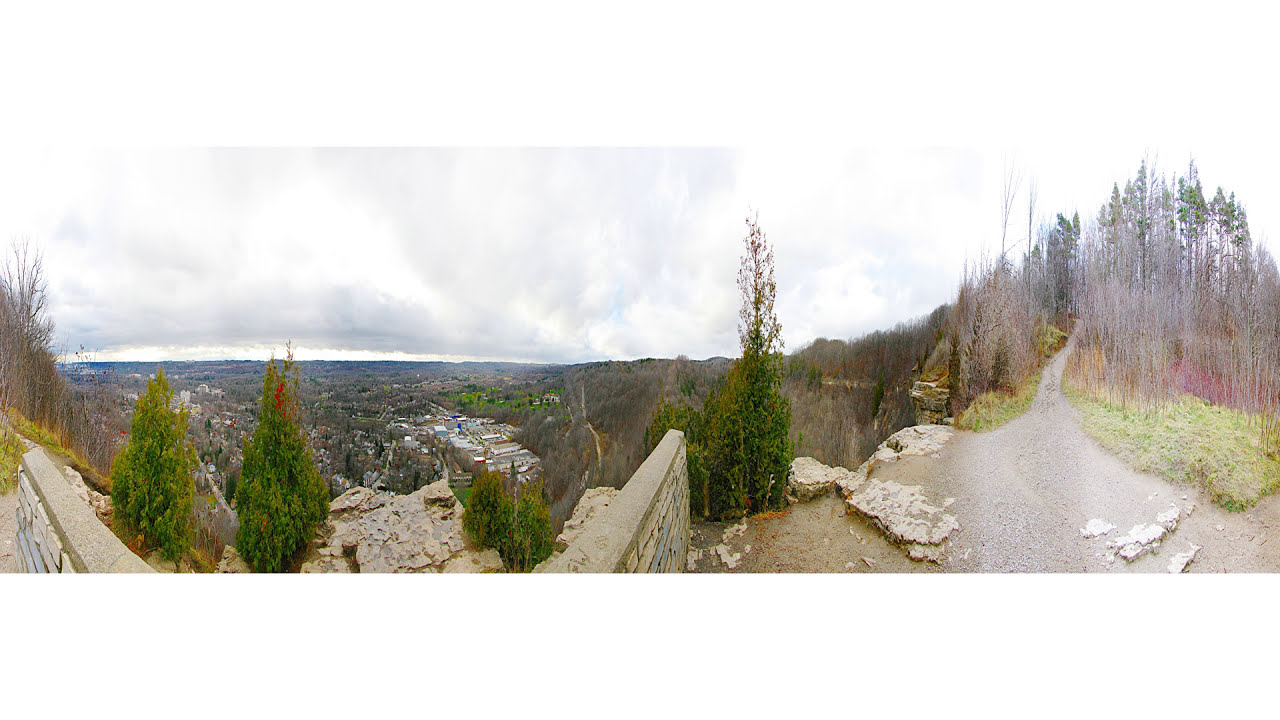This panoramic color photograph captures a stunning view deep in nature, atop a rugged mountaintop. The landscape orientation reveals a sweeping perspective: on the left side, a short stone wall overlooks a valley peppered with rooftops, hinting at nearby civilization. Cypress trees and lush green vegetation, including grass and shrubs, add vibrant color to the scene. To the right, the image transitions to a craggy hillside adorned with both evergreen and deciduous trees, some of which are shedding their leaves. A narrow, dry path meanders through this section, inviting the viewer's eye into the woods and away from the camera. The sky above is mostly white with clouds, suggesting a pleasant day without imminent rain. Despite the serene setting ripe for hiking, the photo lacks any presence of people or animals, emphasizing the tranquility and undisturbed beauty of this natural vista.